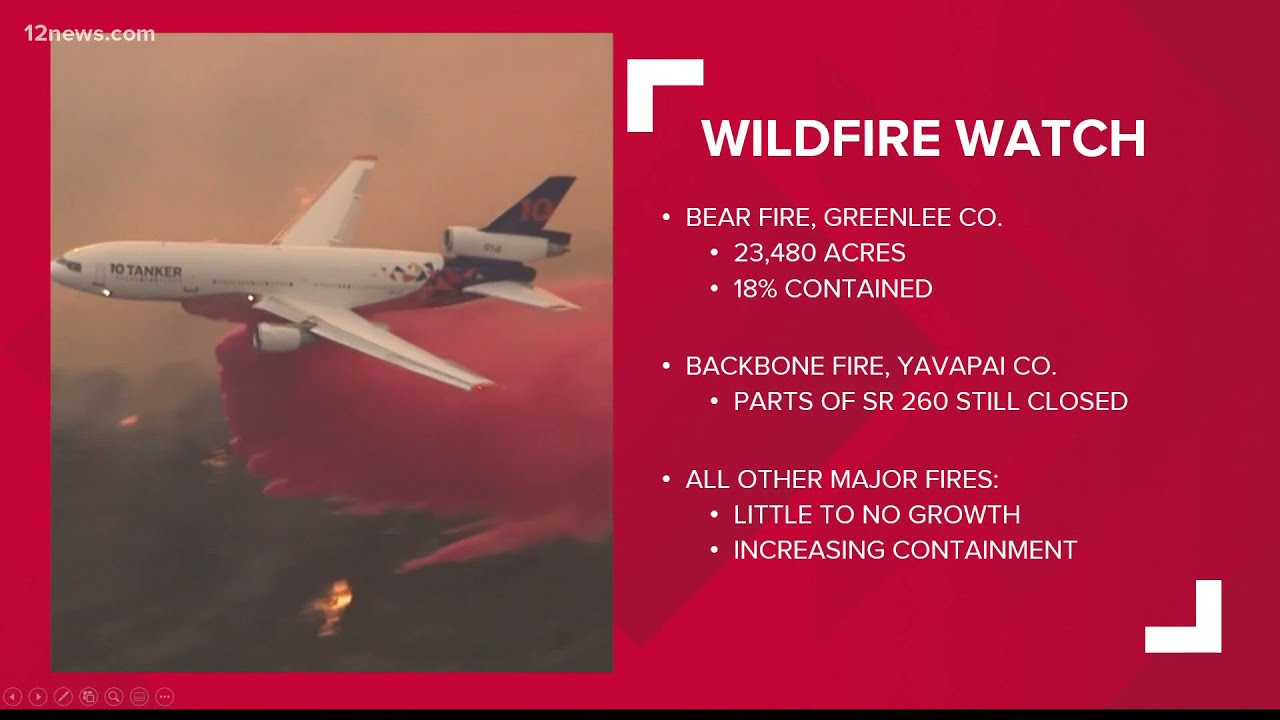The infographic appears as a horizontal, rectangular image set against a dark red background. In the upper left corner, there is a small white font text reading "12news.com." Dominating the left side of the infographic is an image of a large white jet labeled "10 Tanker," with a number "10" on its black tail. The jet is releasing a massive red cloud of fire retardant over a smoky, flame-filled area below, likely battling a wildfire. The sky transitions from a dark gray at the bottom to a reddish hue at the top, heightening the dramatic effect. On the right side, white all-caps text reads "WILDFIRE WATCH." Below this, there are three bullet points detailing current wildfire incidents: "Bear Fire, Greenlee County: 23,480 acres, 18% contained," "Backbone Fire, Yavapai County: Parts of SR 260 still closed," and "All other major fires: Little to no growth, increased containment." The stark contrast of the red background and white text, along with the jet's vivid action, convey an urgent and informative visual related to ongoing wildfire containment efforts.